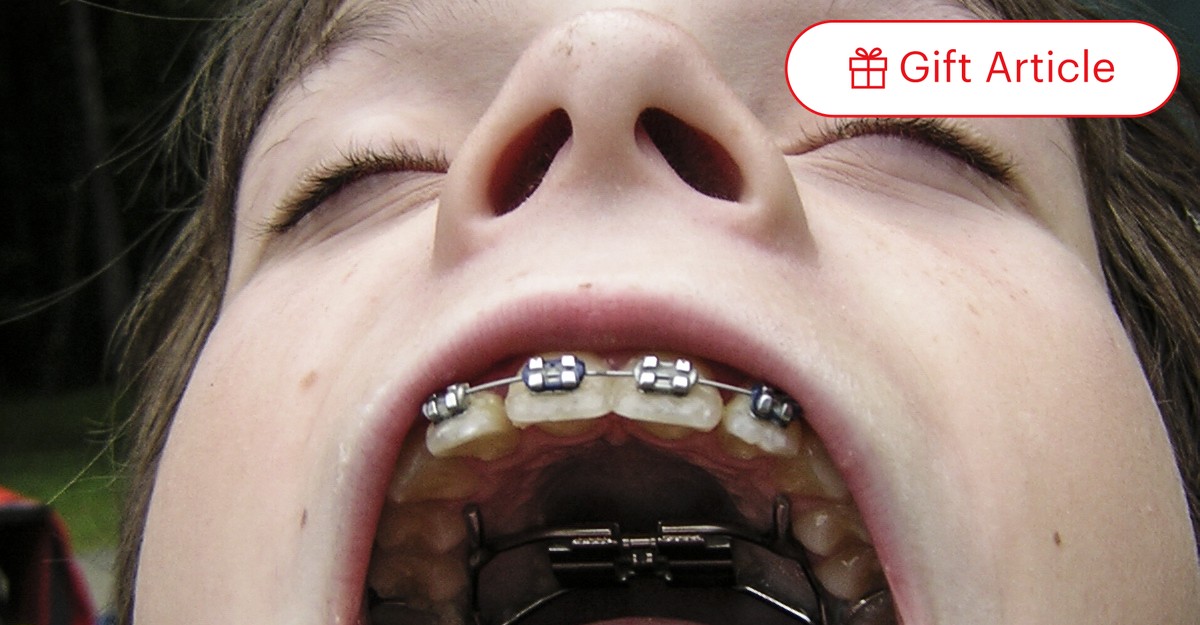The image is a close-up of a person, likely a boy, with closed eyes, brown hair, and multiple moles on their face. The perspective is from mouth level, capturing the extensive metal braces on their upper teeth and a large metallic structure interlocking the teeth along the maxilla. The photograph also reveals the person's nostrils. The background is blurry and not clearly distinguishable. To the top right of the image, there is a white label bordered in red, with a red "GIF" icon next to the text "gift article." Additionally, there is something green visible on the bottom left.